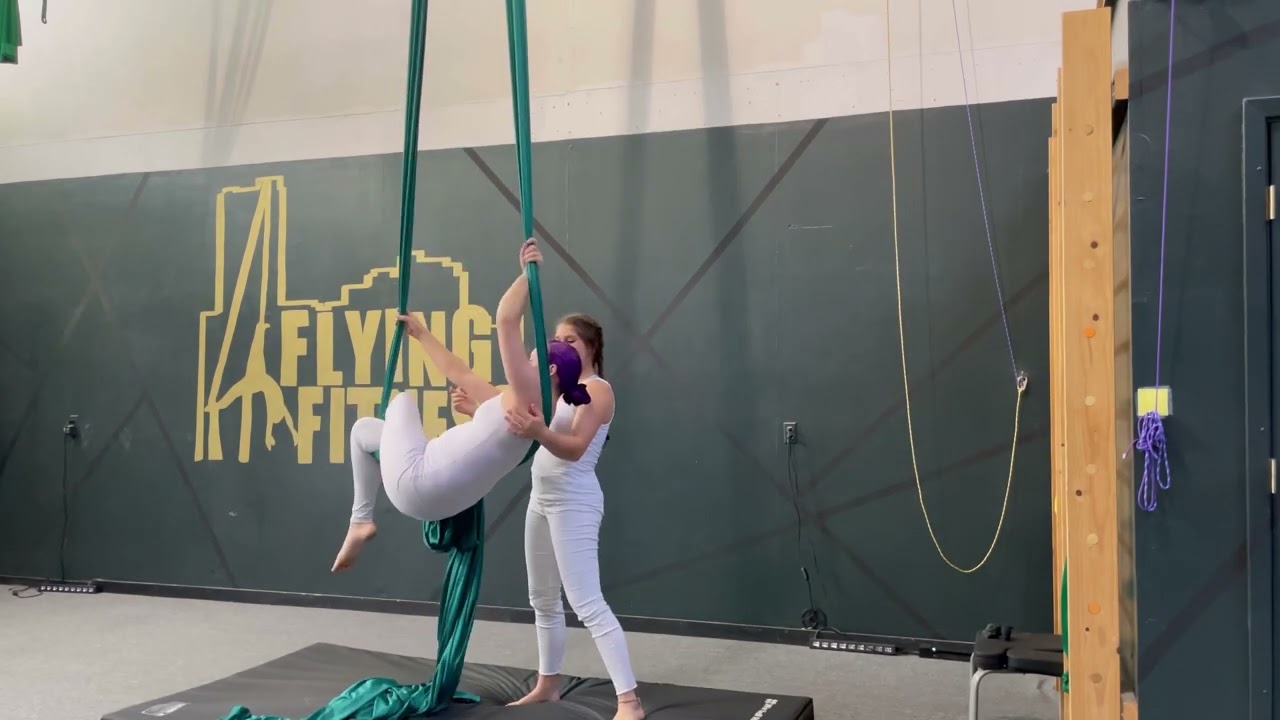The image captures two young gymnasts in a gymnasium, engaging in a balancing act involving aerial silk fabric. The gym features a beige upper wall and a military green lower wall, adorned with a yellow "Flying Fitness" graphic that includes an illustration of an upside-down person on aerial ribbons. The gymnasts, dressed in matching white leotards and tank tops, are performing on a turquoise piece of silk fabric that hangs from the ceiling. One gymnast, with purple hair, is wrapped around the fabric, her right leg supporting her weight while her left leg crosses over it. She uses her right arm to grip the fabric, maintaining her balance, while her friend, with brown hair, assists her by holding the fabric steady. They are positioned over a brown sponge mat placed on a white cement floor for safety. The scene also includes glimpses of brown wood posts to the right and a partially visible doorway, enhancing the gym's busy and functional atmosphere.